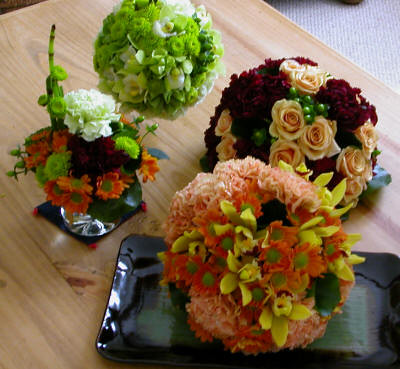This image showcases a beautifully arranged light blonde wooden tabletop, likely made of oak. On this table, there are four artfully crafted bouquets. The bouquet closest to us sits on a black porcelain or ceramic tray, featuring a mix of large, fluffy pink and yellow flowers, alongside some green leaves. Next to this, there's a smaller floral arrangement in a glass, resting on what seems to be a black napkin. This bouquet has an elegant white carnation at the top, accompanied by a dark red flower, and a variety of tiny orange daisy-like flowers interwoven with green buds. Towards the upper corner of the table, there’s a spherical bouquet dominated by green blooms. Another striking arrangement showcases deep red and light pink roses set against a backdrop of green leaves. The combination of these contrasting and complementary colors makes the set-up particularly eye-catching. Surrounding the table, a light gray rug can be seen, along with glimpses of table or chair legs, adding to the cozy, refined ambiance of the scene. These lush, vivid floral arrangements create a beautiful and inviting display.